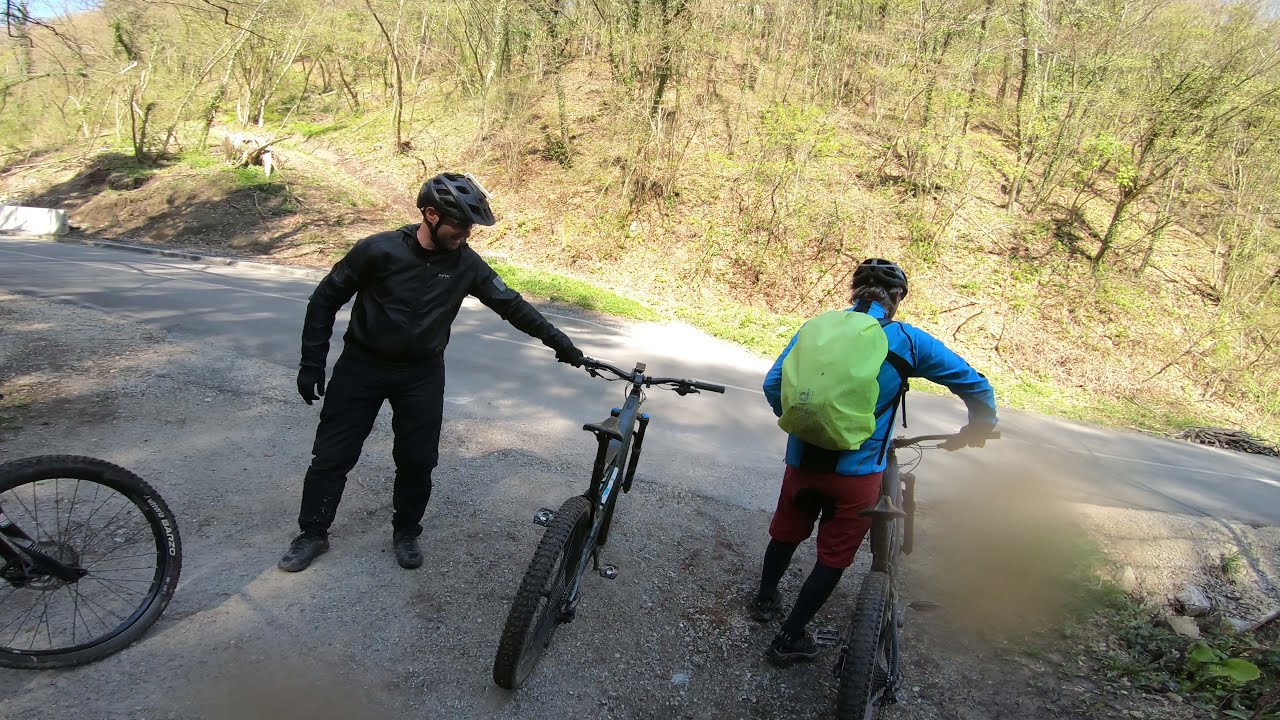In this image, set in what appears to be late fall, winter, or early spring, two men are preparing for a mountain biking adventure on the side of a paved country road, with the faint presence of a third cyclist indicated by the front wheel of another bike poking out from the far left corner. The man on the left is fully dressed in an all-black outfit, including a black helmet, gloves, pants, jacket, and shoes, with his left hand resting on the handlebars of his bicycle. The man on the right brings a splash of color with his aqua blue shirt, light green backpack, red shorts, and long black stockings, along with black shoes that resemble hiking boots. He stands beside his bike with both hands on the handlebars, ready to embark on the ride. Encompassing them is a semi-bare, mountainous background with scrubby, mostly bare trees, hinting at a transitional season. The wooded area across the street enhances the rugged, outdoor setting of their upcoming expedition.